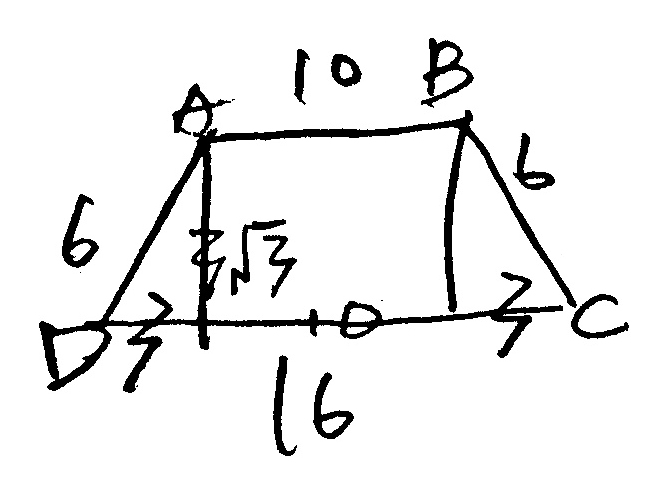In the image against a white background, a complex equation is depicted in black ink. The central figure resembles an abstract structure, somewhat like a tent, composed of a combination of geometric shapes and symbols. 

The primary shape includes a V-like structure intersected by a vertical line topped by another line, alongside an upside-down V with a connecting horizontal line underneath. In essence, it forms a diamond or parallelogram shape intersected in the middle with an extension upwards and downwards.

The vertices of this abstract structure are labeled as follows: 
- **A** at the top-left corner,
- **B** at the top-right corner,
- **C** at the bottom-right corner, and 
- **D** at the bottom-left corner.

Numeric values flank the edges:
- The left side is marked with a 6,
- The top is labeled with a 10,
- The right side also shows a 6,
- The bottom carries a 10, and
- The central vertical section is annotated with 16.

At the two extreme ends of the figure, there are what appear to be squiggly symbols resembling an open three or a stylized Z with an additional line. Located approximately halfway along the vertical line within the central structure, another set of squiggly lines terminate in arrows, followed by additional squiggles and symbols similar to the earlier three-like figures. 

The intricacy of the image suggests a mathematical or geometric problem with a unique set of symbols to represent specific components or relationships within the structure.